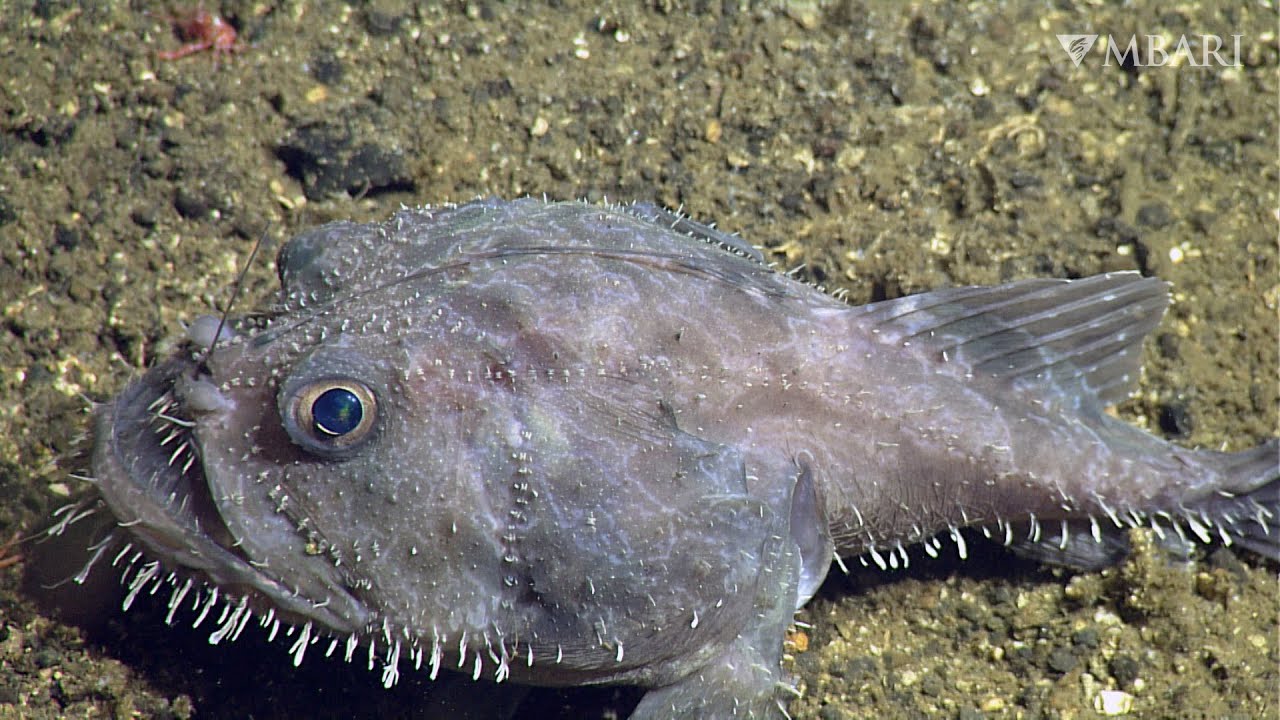In this image, we see an extremely close-up side view of a fish that is situated on dry land. The fish exhibits a striking blend of dark gray and light purple hues. Its blue eye is prominently visible, and a singular gray antenna extends from the left side, near its mouth. The fish features multiple small white lines on its underside, possibly representing its scales or skin texture. Towards the right end of the fish, you can see its fins and tail. The ground beneath the fish is a light brown, rocky terrain. In the top-right corner of the image, there is a logo featuring the acronym "MBARI" accompanied by a triangle symbol to its left.